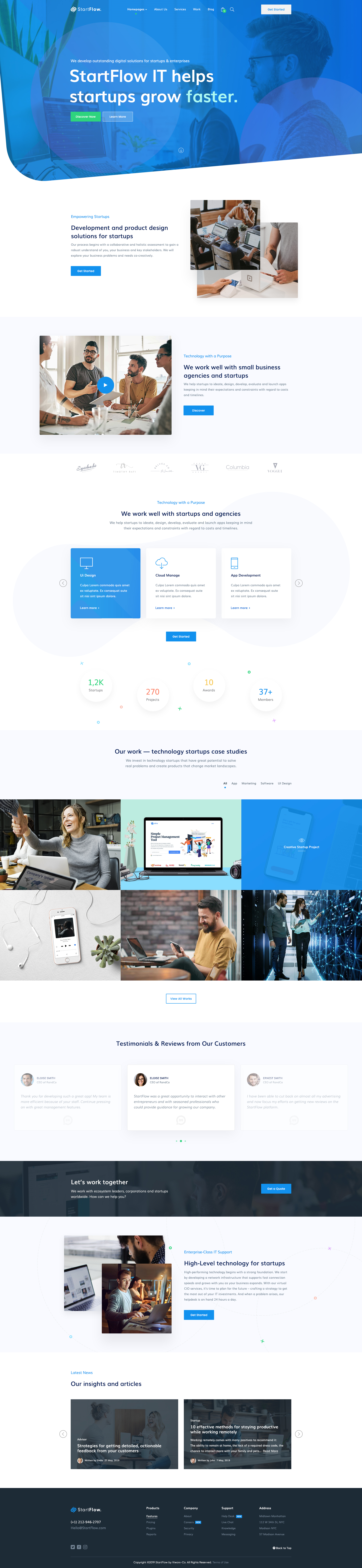The image is a comprehensive screenshot of a website dedicated to technology and computer services, particularly aimed at aiding startups. The header prominently displays the brand name "Start Flow" alongside the tagline "IT helps startups grow faster," emphasizing the site's focus on accelerating business growth through technology. A partially obscured background image depicts a man, with another person faintly visible, both of whom are slightly covered by the overlaid text. Below this header, the page features several descriptive sections arranged in card-like formats, providing detailed information. Stock photos of people in relaxed, seated positions are interspersed throughout the page, further illustrating the targeted user experience.